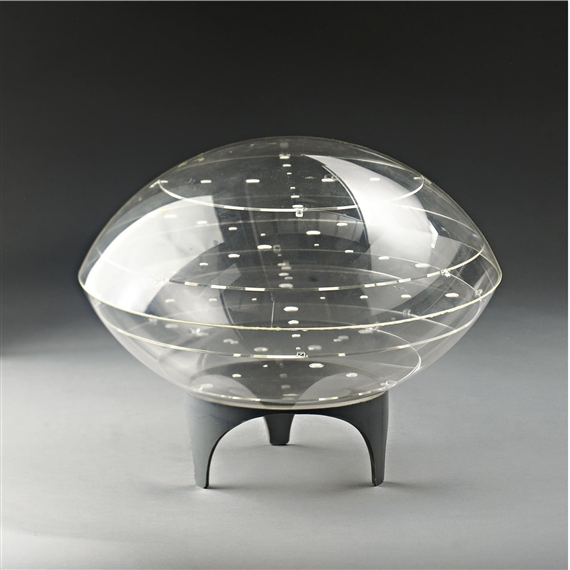This is a vertical rectangular photograph of a striking, artfully crafted sculpture created by Gregorio Vardenego. The centerpiece of the image is an unusual, transparent object that resembles a spacecraft or a pair of conjoined bowls. This clear plastic or glass structure is adorned with white spirals and lines that create a dynamic pattern around its oval, almost flying saucer-like shape. The intricate design includes glittery rings and dashes, adding to its ethereal appearance. This intriguing object sits upon a small, three-legged pedestal, which features half-arch connectors between the legs, giving it a distinctive, modern aesthetic. The surface it rests on is a softer gray color while the background transitions into a dark, charcoal gray, enhancing the prominence of the sculpture. The upper part of the object appears shiny, suggesting the presence of an overhead light source illuminating the artwork and creating subtle reflections and depth within the transparent material.